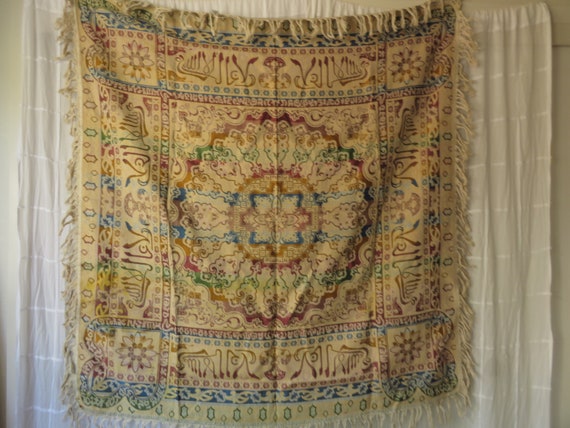A photograph showcases an ornate textile, possibly a scarf or shawl, in a soft, creamy tan or pale yellow color. The textile, which is a square shape with fringed edges, hangs against a sheer white curtain with a darker white wall backdrop, creating a delicate contrast. The centerpiece of the cloth is a vibrant medallion, adorned with a star and surrounded by various colors including yellow, red, blue, and purplish hues. Hieroglyphic-like writing or foreign characters decorate all four sides of the square, with additional floral designs gracing each corner. The designs also feature banners between the flowers and an intricate combination of reds, dark reds, browns, oranges, and yellows, making it a rich and detailed piece of fabric art. The top and bottom borders are highlighted with a medium blue stripe, followed by a yellow one, adding an elegant frame to the entire textile.